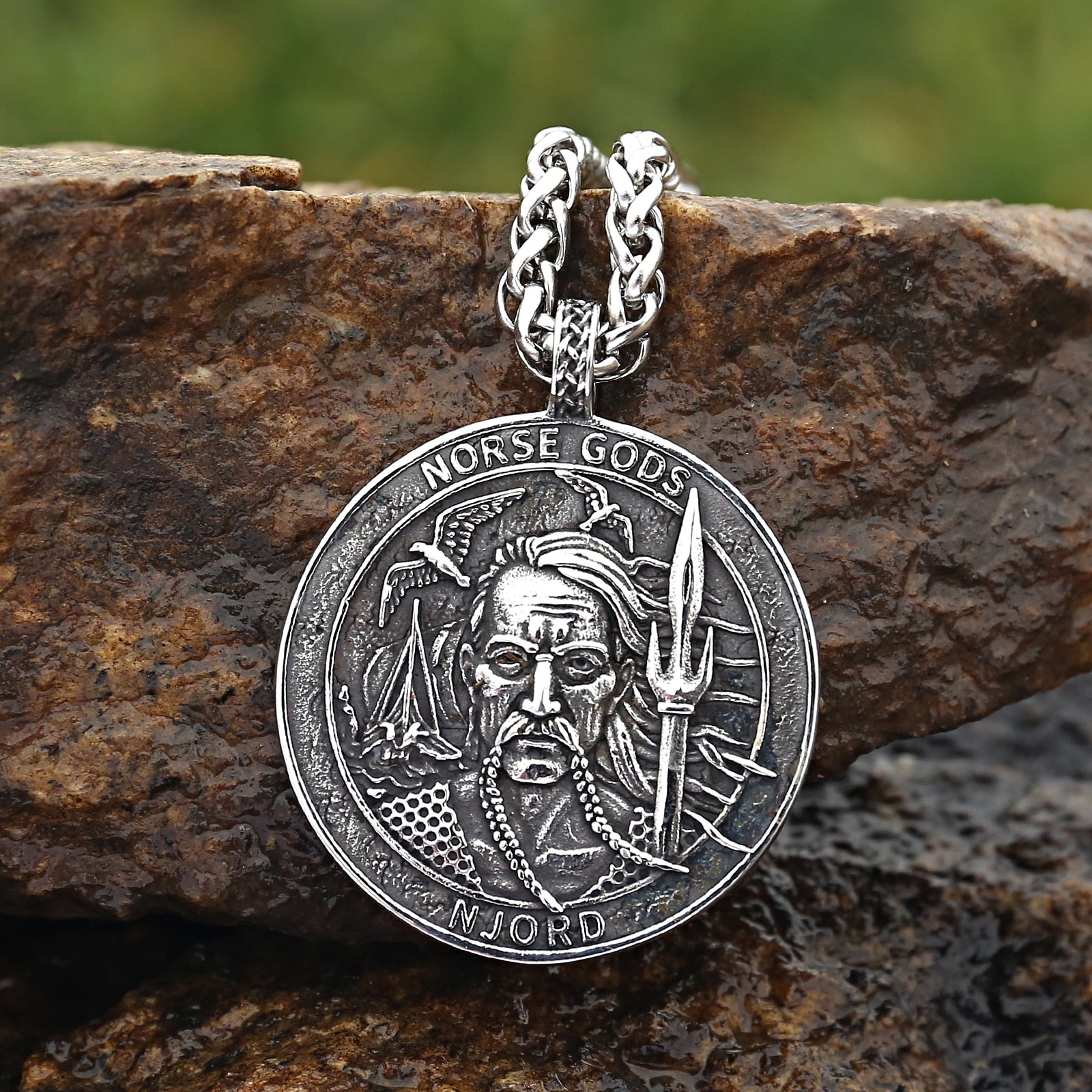This detailed photograph, taken outdoors during the daytime, showcases a circular silver medallion hanging from a chrome chain draped over a wet, reddish-brown rock. The background is blurred with tones of green, suggesting a natural, outdoor setting. The medallion, which appears to be approximately six inches in diameter, features an intricate design centered around a Norse deity named Njord, as indicated by the inscription "Norse gods" at the top and "Njord" at the bottom of the outer circle.

In the center of the medallion, Njord is depicted with a long, braided mustache, his hair blowing to the right as though caught in a gust of wind. Njord's defined features include a straight nose, broad eyebrows, and almond-shaped eyes, and he is seen looking directly at the viewer. He holds a spear in his right hand, symbolizing his divine authority and warrior prowess. Additionally, Njord is adorned in a metal mesh armor, emblematic of his strength and valor.

The scene around Njord includes two birds in flight, reminiscent of seagulls, and a Viking ship with a prominent sail, reinforcing the maritime connections associated with the Norse god. The craftsmanship of the medallion and its detailed imagery evoke a strong connection to Norse mythology and its legendary figures, making it a captivating piece of wearable art.